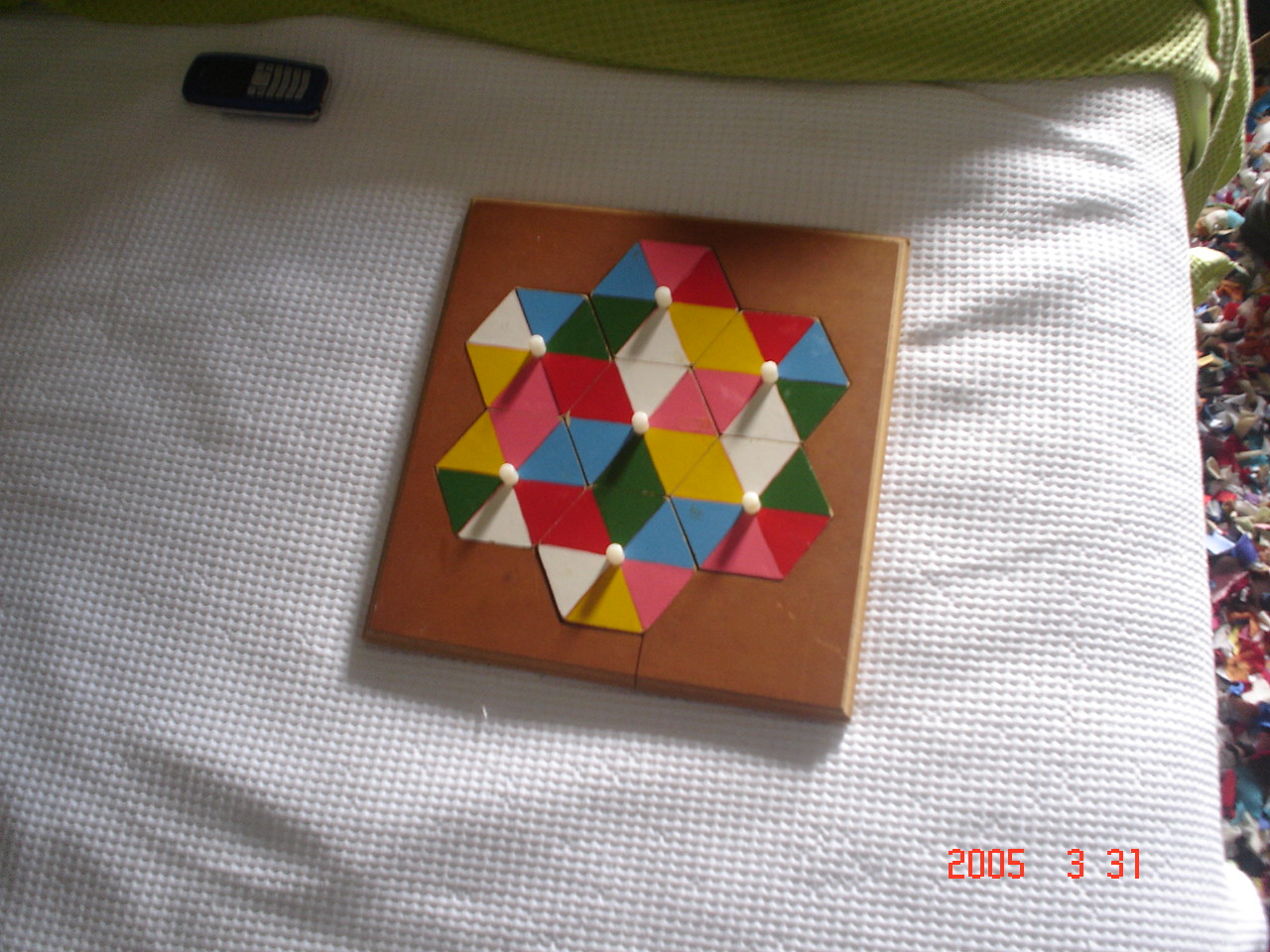The image captures a detailed and somewhat nostalgic scene set on a bed with white, dotted sheets and a green blanket at the top. Dominating the center is a wooden toy or puzzle board made from brown wood, featuring six colorful triangular pieces—each one either green, blue, pink, red, yellow, or white—forming a larger hexagonal pattern. Each piece is secured in place by white pins. In the top left corner of the image, there's an old Nokia-style smartphone with a blue body and white keys, resting by a set of keys. To the right, a narrow strip of the floor is visible, cluttered with various colorful shapes and what seems to be trash. The bottom right corner of the image is marked with a red timestamp reading "2005 331."